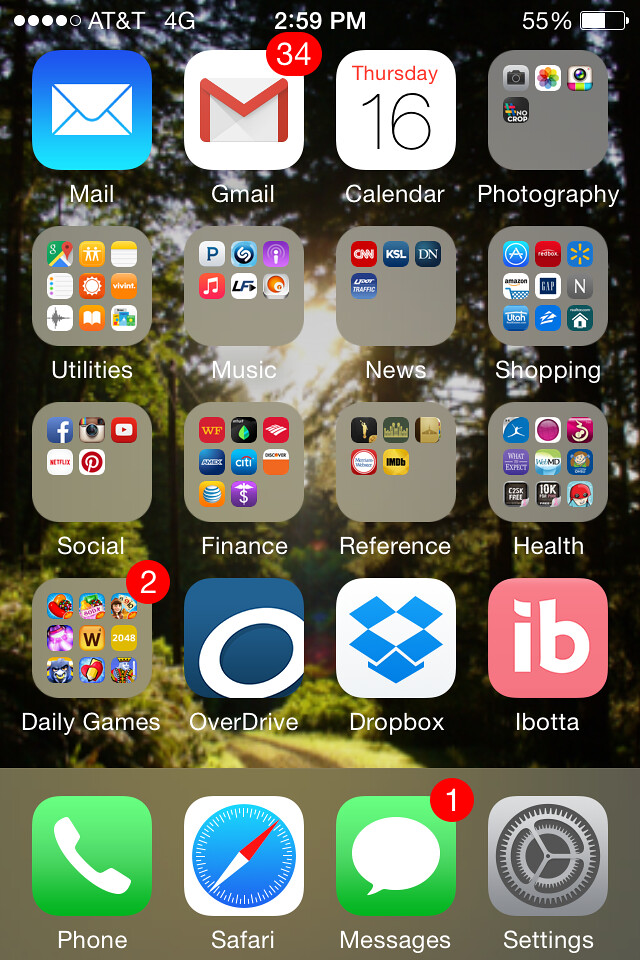A detailed photograph of an Apple iPhone home screen reveals various apps and widgets. At the bottom of the screen, from left to right, are the Phone app, Safari browser, the Text Message app displaying one unread message, and the Settings app. The phone's battery is at 55%, and the time is 2:59 PM. The device has 4G service with AT&T, showing four bars of signal strength.

In the top left corner of the home screen, the Outlook Mail app is visible, followed by the Gmail app with 34 new emails. The date, Thursday the 16th, is displayed on the Calendar app. There is a Photography folder containing the Camera app, Photos app, and two other unidentified apps.

The Utilities folder includes Google Maps, People, Vivint, Voice Memos, Notes, and Tasks. Additionally, there is a Music folder housing the Apple Music app. Other visible app categories are News, Shopping, Health, Reference, Finance, Social, Daily Games, OverDrive, Dropbox, and Ibotta.